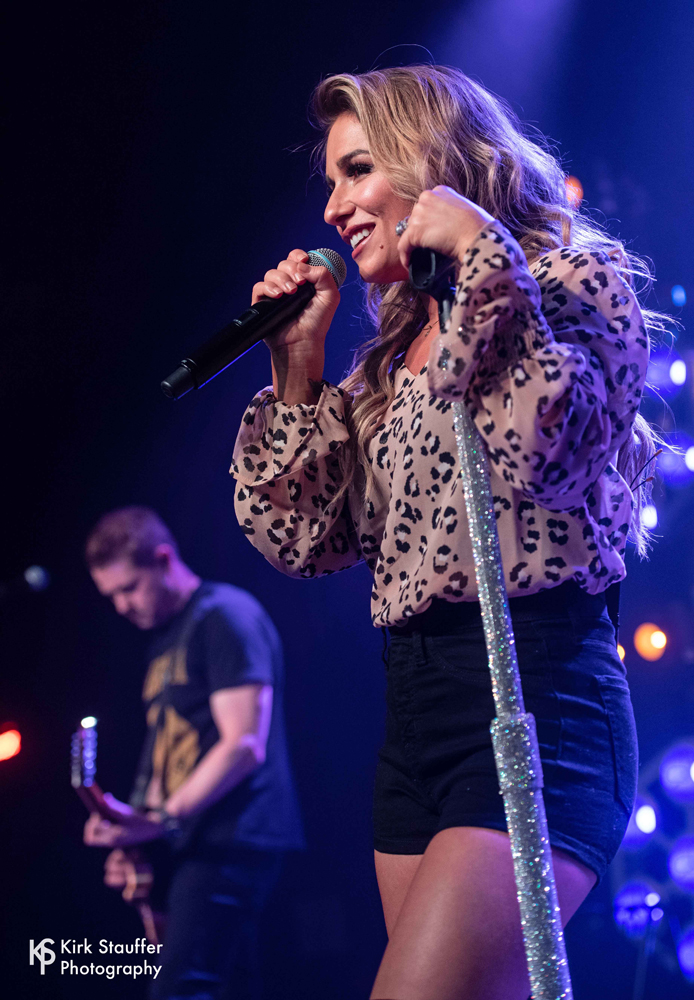This photograph captures a live stage performance featuring a young female singer, likely in her 20s, who is believed to be Deborah Gibson, a renowned 80s teen singer still performing. She is the main focal point, holding a microphone in her right hand and leaning on a sparkly mic stand with her left hand. Her long, brown hair with blonde highlights cascades down her back. She is dressed in a leopard-print blouse with loose sleeves tucked into black shorts, revealing her legs. The backdrop is mostly dark, punctuated by yellow, white, and blue stage lights creating a dramatic effect. To her left, there is a guitarist with short brown hair, wearing a black T-shirt with yellow writing, engrossed in playing his instrument. The bottom left corner of the photograph bears the watermark "Kirk Stauffer Photography" in white text.